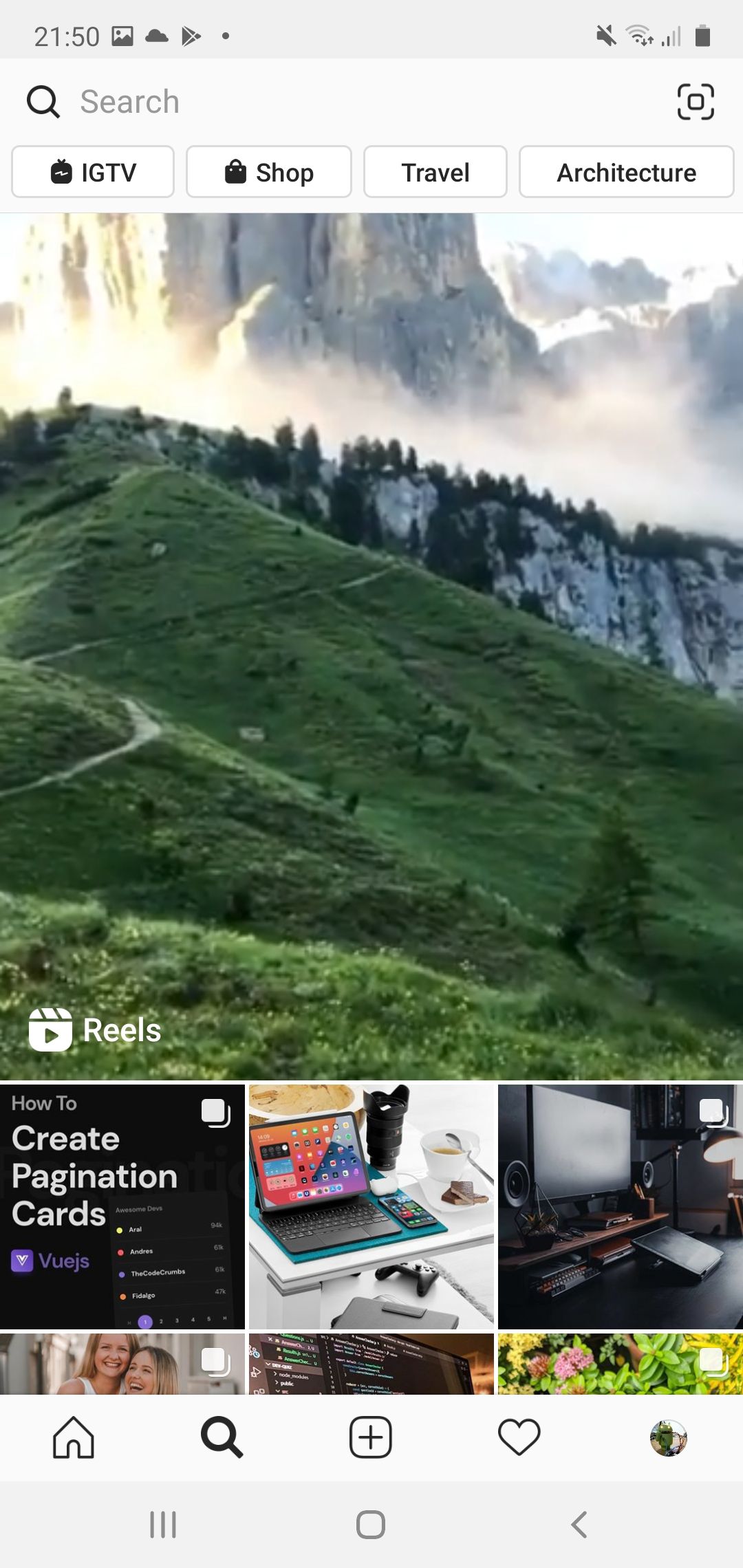This image is a screenshot of someone's smartphone interface. In the top left corner, it displays the current time as 21:50. Adjacent to the time, there's a series of symbols: a square resembling a picture icon, followed by a cloud symbol, and a side-turned triangle. The top right corner shows a nearly full battery icon. Moving left from the battery icon, there's a symbol indicating WiFi signal strength with two bars, another signal strength icon also showing two bars, and a sound symbol crossed out with a diagonal line indicating the phone is on silent mode.

The central focus of the image is a photograph depicting a lush, green, grassy hill. Positioned in the upper half of the screen, there are rectangular tabs labeled IGTV, Shop, Travel, and Architecture. At the very bottom of the screen, there are additional text and images. One of the boxes reads "how to create pagination cards," and to its right, there's a red box featuring an image of a laptop.